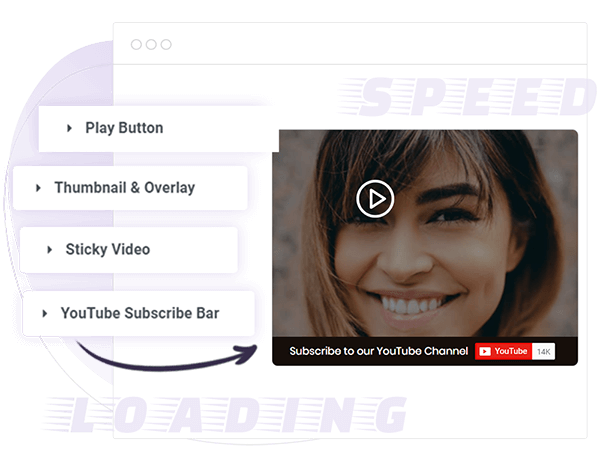The image features a dynamic multimedia layout with various graphical and textual elements. At the top, three circles are prominently displayed over a white background. To the right side of the image, the word "SWEET" is written in grey letters, accompanied by stylized lines suggesting motion behind each letter, spelling out "S-P-E-E-D."

On the left side of the image, a series of multimedia controls are shown: a "speed" indicator, a play button, a thumbnail and overlay, a sticky video option, a YouTube subscribe bar, and an arrow pointing to the right. 

At the bottom of the image, there is a loading bar accompanied by dialogue marks such as L, L-M-R-X-O, L-M-R-X-A, L-M-R-X-T, L-M-R-X-I, L-M-R-X-N, and L-M-R-X-T, suggesting different states of loading or buffering.

Overlaying the entire image is a semi-transparent shadow, with a play button superimposed in the center. A woman with short hair, white teeth, and thick eyebrows is featured, possibly the subject of the video. 

The background of the image is mainly white but transitions to purple on the left side, where the letters are also rendered in purple. Four rectangles are arranged vertically at the top with varying levels of indentation; the first rectangle is indented while the second one is positioned lower.

The overall scene suggests a screenshot or graphical representation of a multimedia interface, likely related to a video or streaming platform.